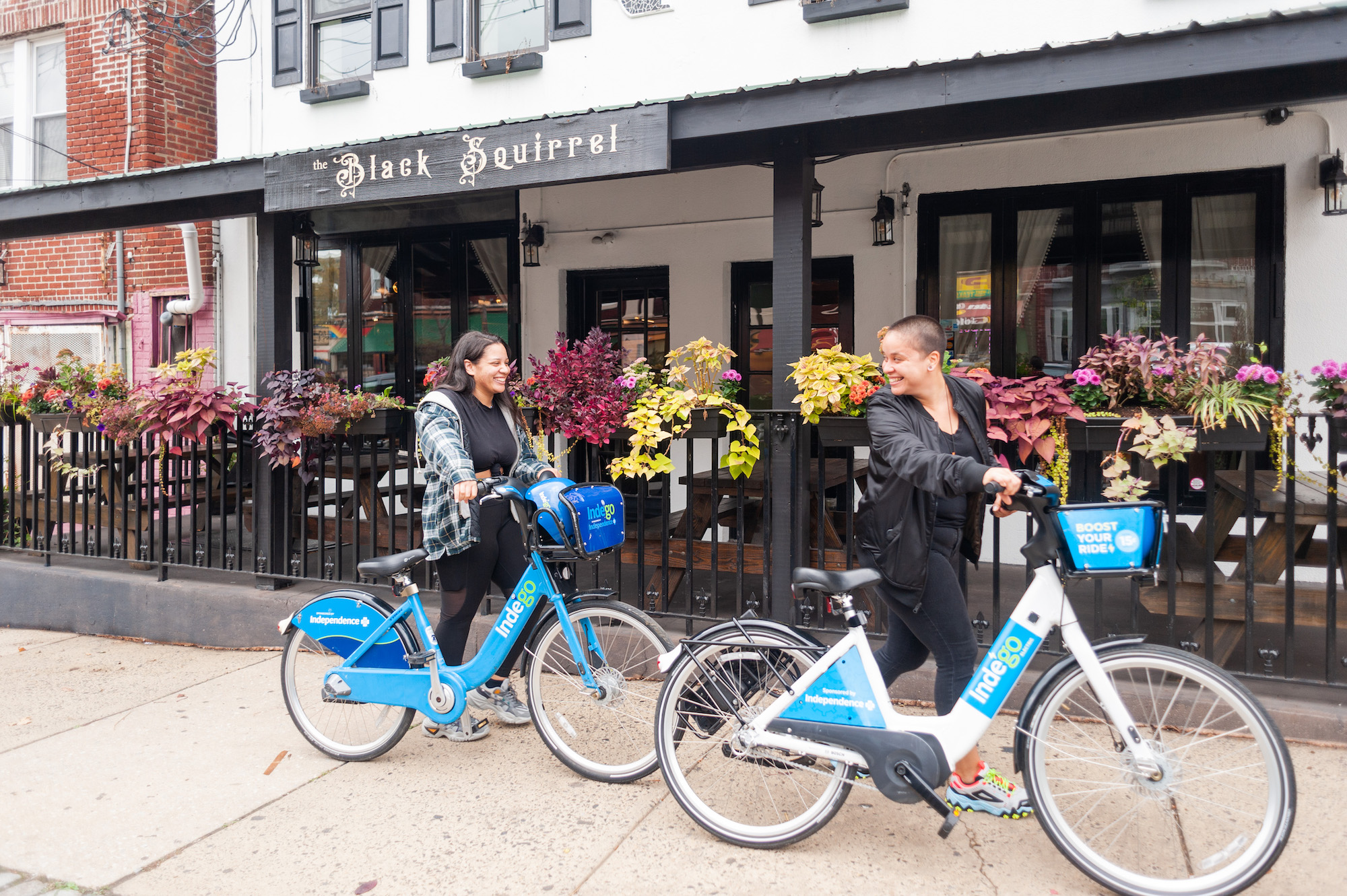In this outdoor photograph, two individuals are seen walking their blue and white rental bikes, branded with "Indigo," along a sidewalk in front of a cafe named "The Black Squirrel." The person in front, who has closely cropped dark hair, is dressed in all black with a jacket over a black top and is turning their head to look back at their companion. The second person, with long shoulder-length dark hair, is wearing black tights, sneakers, a black top, and a plaid hoodie jacket. Both individuals appear to be in good spirits, smiling and engaging with each other as they push their bikes. They are walking past a black fence adorned with planters filled with various plants and flowers, and nearby is a brick-red building with additional foliage visible. The scene captures a moment of camaraderie and urban charm against the backdrop of a quaint downtown area.